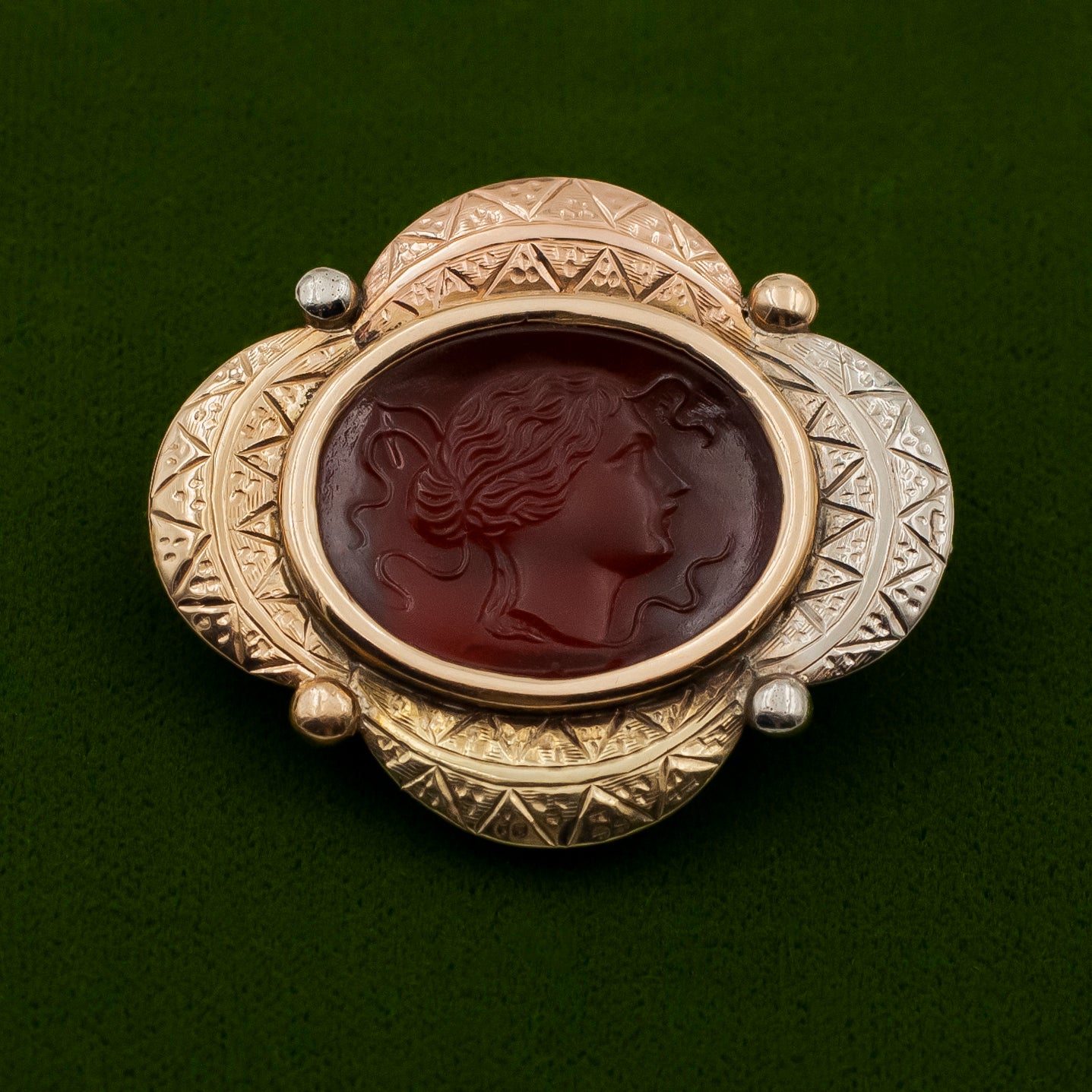This photograph depicts a delicate artifact, believed to be a brooch, set against a richly textured dark green velvet background. The brooch, made of silver or a light gold metal, displays intricate craftsmanship with an ovular design consisting of four interconnected arches — one each at the top, bottom, left, and right. Each arch features fine etchings with vertical lines and small dots, interconnected by a detailed band that encircles the entire piece.

At the center of the brooch is a prominent brown coin or medallion, which appears to hold a red wax stamp. This stamp bears the detailed engraved image of a young woman with her hair tied back into a bun, with a few wisps of hair escaping her coiffure. The woman is depicted in profile, facing left, with a sharp nose and a strong jawline, giving a dignified and classical impression. This elegant piece of jewelry combines intricate metalwork with a classical portrait, capturing the essence of detailed and skilled craftsmanship.